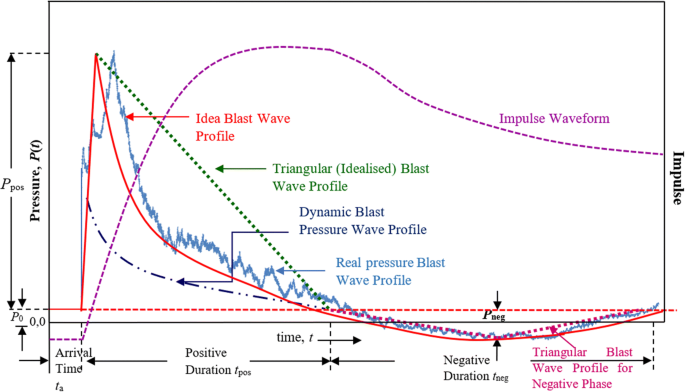The image depicts a detailed graph chart on a white background, focusing on various blast wave profiles. On the left side, "Pressure (P)" is labeled prominently with arrows pointing up and down. On the right side, "Impulse" is highlighted in bold black letters. The graph also features the terms "Triangular Idealized Blast Wave Profile," "Dynamic Blast Pressure Wave Profile," and "Real Pressure Blast Wave Profile" spread across it.

The horizontal axis is marked with labels such as "Arrival Time," "Positive Duration (t_POS)," and "Negative Duration (t_neg)." The chart includes different colored lines representing various wave profiles: a solid red line for the ideal blast wave profile, a dark blue dotted and segmented line for the dynamic blast pressure wave profile, and a blue wavy line for the real pressure blast wave profile. Additionally, there is a pink dotted line that dips downward. 

In red letters, the phrase "Triangular Blast Wave Profile for Negative Phase" is indicated, while a dark blue dotted line labeled "Impulse Waveform" traverses the graph, providing a comparative measurement. This complex chart visually represents the interplay of different waveforms and their respective pressures and impulses.